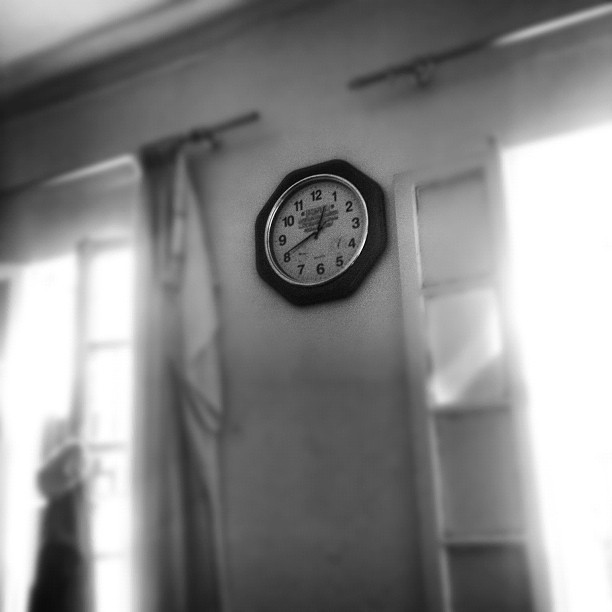The image depicts a striking black and white photograph of an octagonal clock, prominently fixed on a wall. The clock serves as the focal point with its vivid black and white tones that contrast sharply against the muted grayscale surroundings. Positioned between two large windows, each flanked with open shutters, the scene is bathed in natural light streaming through the glass panes, illuminating the area around the clock. The windows are outfitted with glass shutters, one on the left with a curtain and possibly a person faintly visible, albeit blurry, standing by it. The clock itself features bold black numerals from 1 to 12, and has a clear outer hexagonal black shape punctuated by a metal-accented inner circle. Its black hour and minute hands display the time as 12:41, just above unreadable black text situated under the number 12. The overall scene inside the house gives a feeling of focus on the clock, with other elements subtly blurred, drawing attention to the meticulous details of the timepiece.